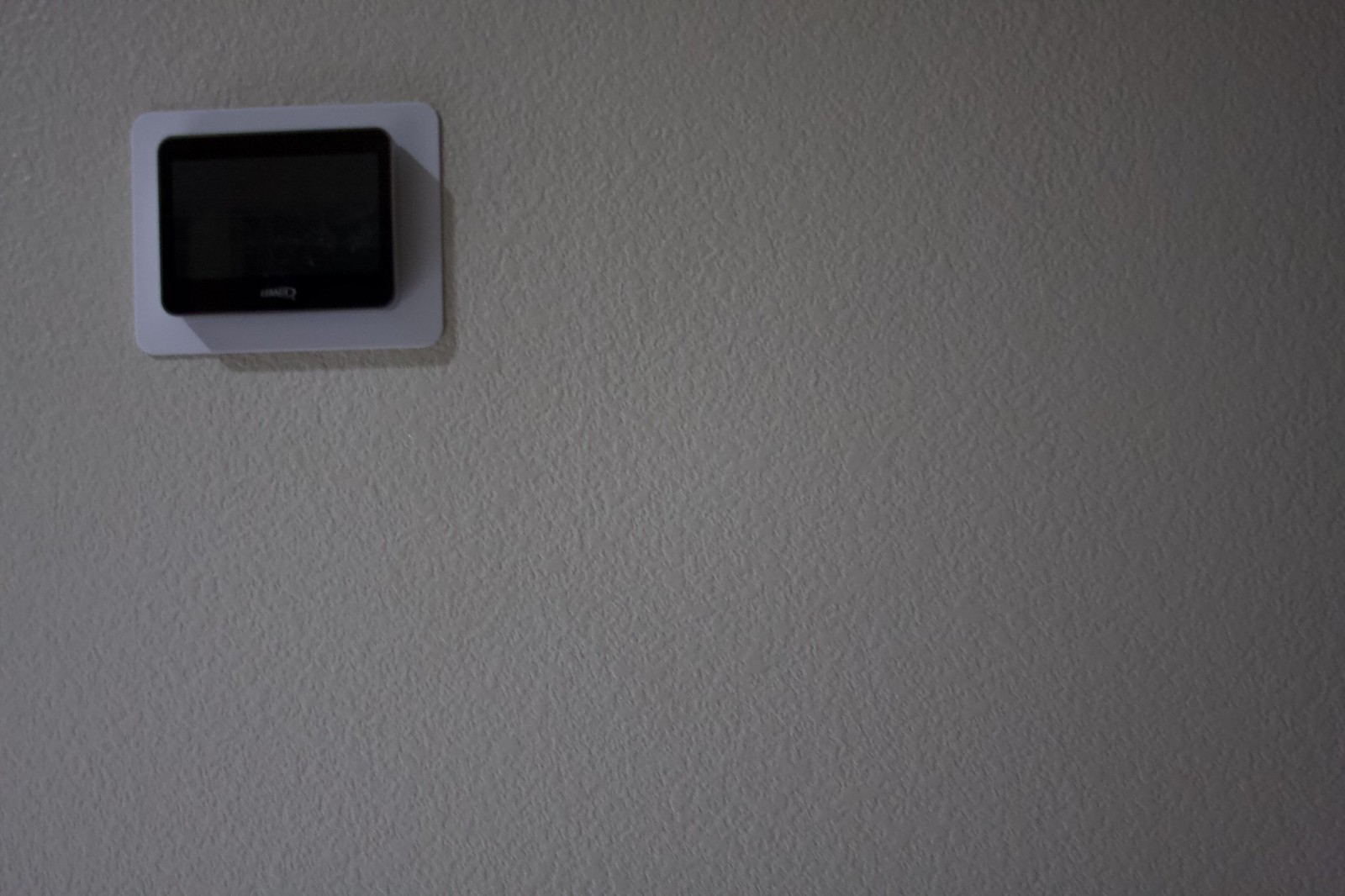The image features a textured white wall with a prominent electronic device mounted in the upper left-hand corner. The device is a sleek, black rectangular unit, possibly a digital thermostat, perched on a larger white frame that is affixed to the wall. Though the image is somewhat dark and lacks clear details, the front of the black unit appears to house a screen. Below this screen, text in a gray font likely displays the brand name. The photograph's angle suggests the device is installed on a vertical wall rather than the ceiling.